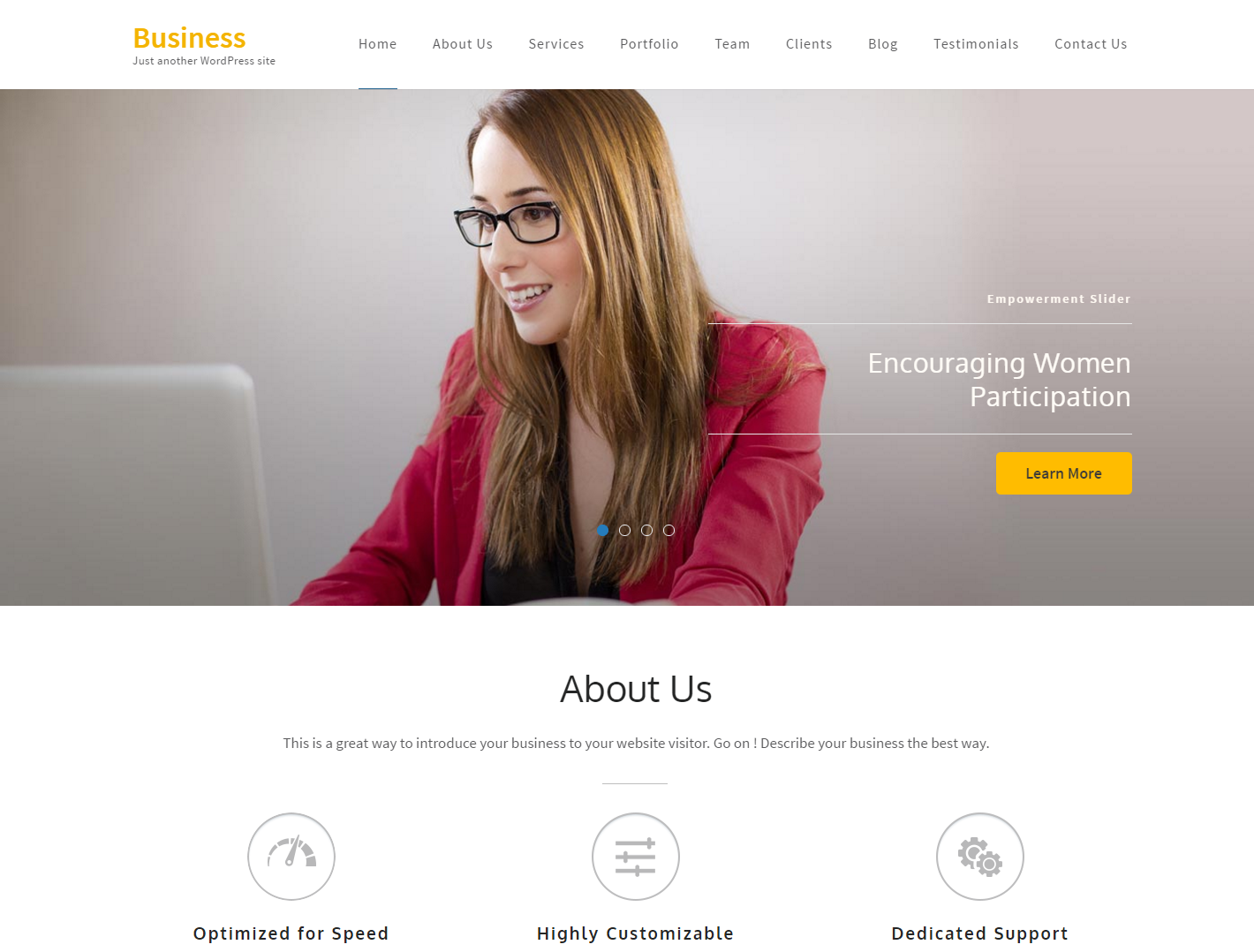In this detailed photographic image, a web address is displayed alongside a structured business website layout. In the top left corner, the word "Business" is prominently featured in a yellow font, immediately catching the viewer's attention. Below, the phrase "Just Another WordPress Site" is written in a dark gray font, indicating a standard WordPress template.

The website's navigation bar is clearly visible and includes the following menu options: "Home," "About Us," "Services," "Portfolio," "Team," "Clients," "Blog," "Testimonials," and "Contact Us." The background of the site is a subtle gray, providing a neutral canvas that accentuates the site's content.

Central to the image, a woman with light brown hair is seated at a computer. She's wearing stylish black-framed glasses and a confident smile as she looks at her computer screen. Her vibrant red blazer adds a pop of color and suggests a professional and energetic atmosphere.

To the right of the woman, bold text reads "Encouraging Women Participation Empowerment," accompanied by a slider button labeled "Learn More," which is set against a yellow background with black font. This section is highlighted to draw attention to a call-to-action.

Further down, the phrase "About Us" is written in black, inviting visitors to learn more about the business. A description follows, encouraging the site owner to effectively introduce their business to visitors.

Additionally, there are three circular icons with text. One circle proclaims "Optimized for Speed," another "Highly Customizable," and a third features a gear icon accompanied by "Dedicated Support." These icons emphasize the website's key features and benefits, ensuring potential clients understand the value of the services offered.